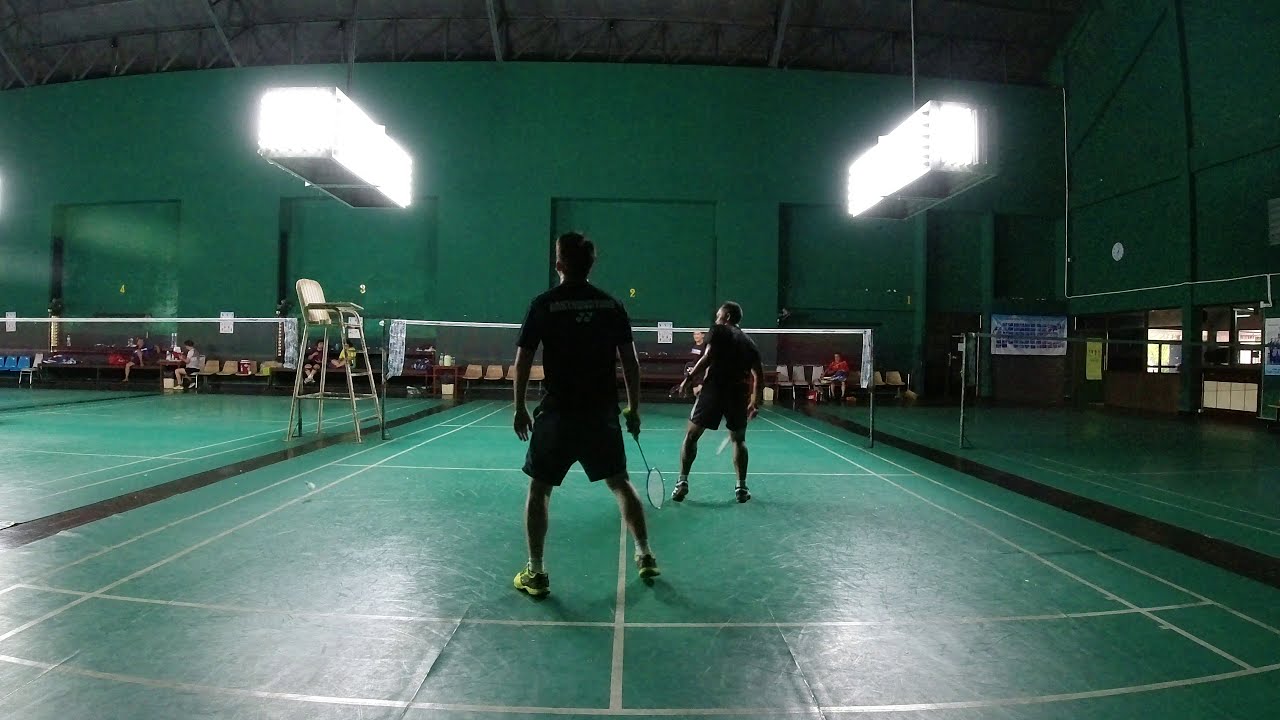The photograph captures an indoor badminton match in what appears to be a recreational center or gymnasium with a greenish hue. The image focuses on a single court, although at least three courts are visible. The walls and court are predominantly green, with other colors like white, black, yellow, red, brown, and blue adding subtle details. Two men, dressed in navy blue shorts and collared shirts, are positioned with their backs to the camera, holding racquets in their right hands, pointed downward. The center of the frame features the net and the badminton birdie, with two bright rectangular bar lights hanging high above. On the left side, an empty umpire chair stands, while two spectators sit on the sidelines. The far side of the net shows another player, partially obscured by the man on the left. Signs in the background are too small to decipher, but they blend into the overall scene without drawing focus away from the match.